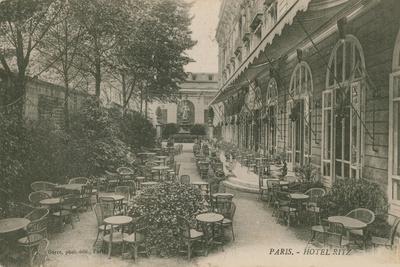This black and white, antique photograph captures the outdoor seating area of the historic Paris Hotel Ritz, likely taken around the turn of the 19th to early 20th century. The view showcases a charming, stone-floored patio lined with café tables and chairs awaiting guests. Lush greenery, including tall trees and green bushes, frames the scene with a picturesque touch, especially along the left side. To the right, the side of the hotel features large, rectangular windows topped with smaller, circular ones, opening out into the serene garden setting. In the distance, another building with an intricately designed roof adds architectural interest. The overall composition, with its faded, grayscale tones, exudes an artistic and nostalgic ambiance.